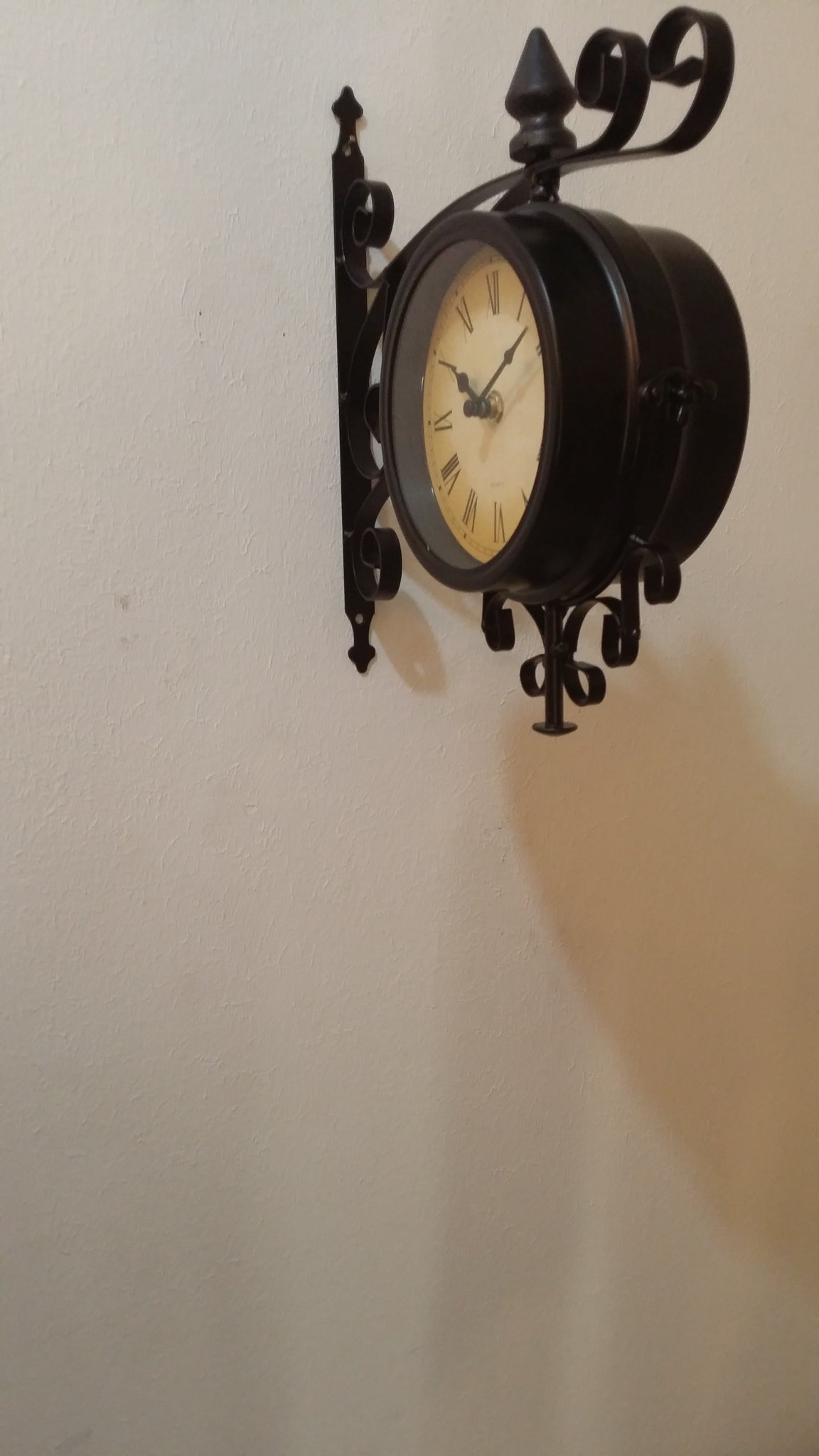This photograph features an ornate black wrought iron clock mounted on a white, slightly grayish wall, casting a shadow to the right and downwards. The clock itself is circular, encased in a sophisticated black metal housing adorned with elaborate curves and intricate designs, including curly elements reminiscent of leaves and a spire-like point at the top. The clock's face is a worn, yellowish-cream color displaying Roman numerals from I to XII, contrasted by thin black hour and minute hands fastened with a silver pin. The time shown is approximately 10:08, with the hour hand on X and the minute hand between I and II.